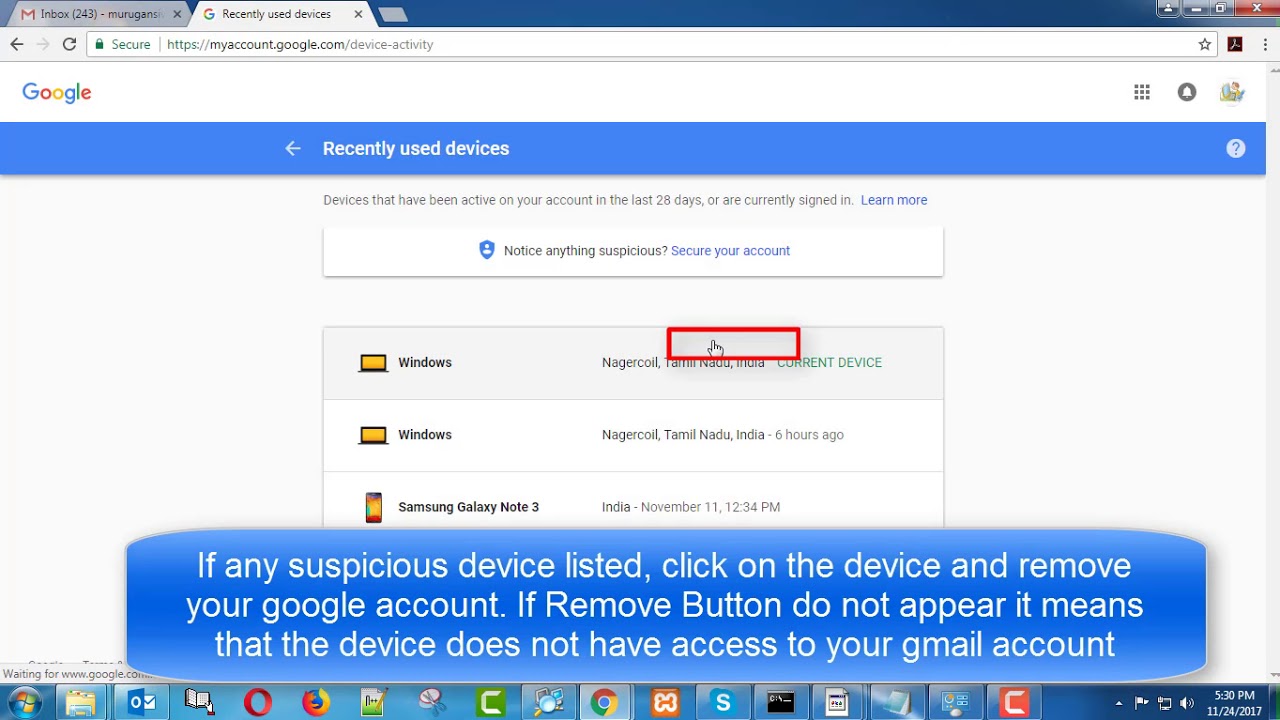A detailed descriptive caption:

---

The image depicts a user's landing page on Google, particularly focusing on the "Recently Used Devices" section. At the very top, a navy blue banner stretches across the screen, showing two open tabs: one for Gmail, revealing the user has 243 unread emails, and another labeled "Recently Used Devices." To the far right of this banner, there are icons for closing, maximizing, and minimizing the window, as well as a people icon. Below the banner, there's a white search bar displaying the URL "https://myaccount.google.com/device-activity."

The main portion of the page is set against a white background, featuring the Google logo in its traditional colors in the upper left. Beneath the Google logo, a prominent bright blue ribbon spans the width of the page, with "Recently used devices" written in white text and a back arrow. To the right of the ribbon, there's a white circle containing a blue question mark for help. 

Immediately below this bright ribbon, in light gray text, it states, "Devices that have been active on your account in the last 20 days or are currently signed in," with a "Learn more" link in bright blue to the right. Further down, there's a highlighted white box stating, "Notice anything suspicious?" followed by a "Secure your account" link in bright blue.

The central content comprises a vertical list of devices that have recently accessed the account. Listed devices include two labeled "Windows" and one "Samsung Galaxy Note 3," all indicating sign-ins from locations in India. Across this list, a wide bright blue banner provides additional instructions in white text: "If any suspicious device is listed, click on a device and remove your Google account. If the remove button does not appear, it means that the device does not have access to your Gmail account."

---